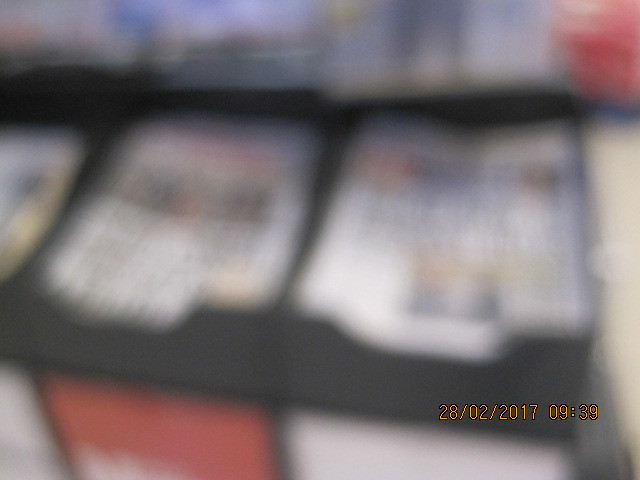This image is a heavily blurred photograph, making it challenging to discern most details. The only clear element is a visible timestamp in the lower right-hand corner, displaying "28/02/2017 09:39." Despite the blur, the image appears to depict a black, metal-framed newsstand or shelf, possibly holding newspapers or magazines due to the visible white rectangular areas that suggest text and headlines. The structure features multiple frames—one predominantly red, and others white. The color palette includes black, red, white, blue, and yellow in various sections.